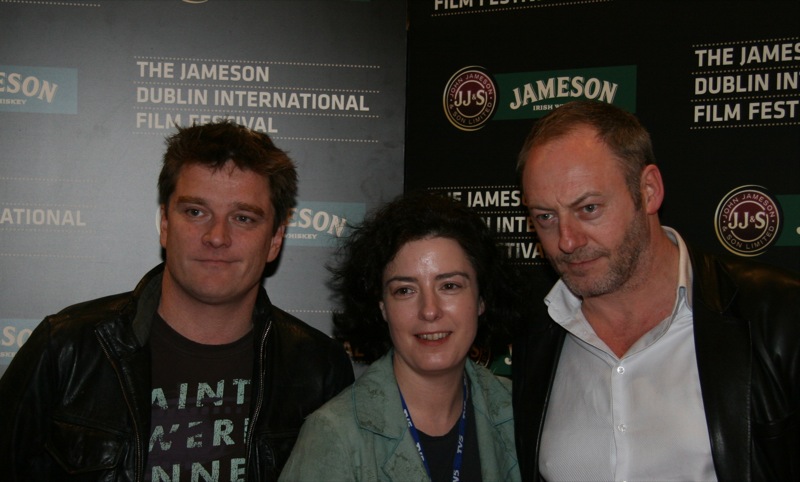In this detailed photograph, we have three people standing side by side, captured from the chest up at the Jameson Dublin International Film Festival. The background is filled with various banners and logos from the event. On the left, a man with short brown hair is smirking softly. He's wearing a black leather jacket over a t-shirt with some text on it. In the center is a woman with dark brown, medium-length hair, smiling gently. She's donning a green jacket over a black t-shirt, with a lanyard around her neck. To the right, a man, likely the famous person in the trio, is dressed in a white button-down collared shirt, left unbuttoned at the top, and a black leather jacket. He has a beard and thinning hair and is also smiling softly. All three individuals are Caucasian, and the setting clearly shows the festival's signature branding.